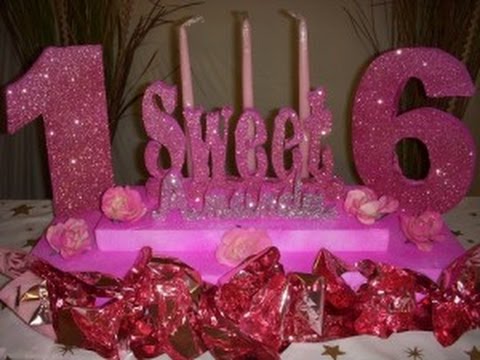The image depicts a detailed table decoration set for a Sweet 16 birthday party. Dominating the setup is a pink base arranged with three white candles, which are unlit and stand in a formation representing the "16"—a '1' on the left, 'SWEET' in the middle, and a '6' on the right. In front of the candles, the name "AMANDA" is delicately written in white, though it's somewhat difficult to discern. Surrounding the pink platform are small flowers, and scattered on the white tablecloth are gold stars enhancing the festive look. In addition, glittery red paper is elaborately draped in front, adding a touch of sparkle. The background includes a pale yellow wall adorned with plants, completing the celebratory ambiance with a harmonious blend of pinks, reds, whites, and golds. An unlit cake is positioned behind the candles, further indicating that the party is yet to commence.